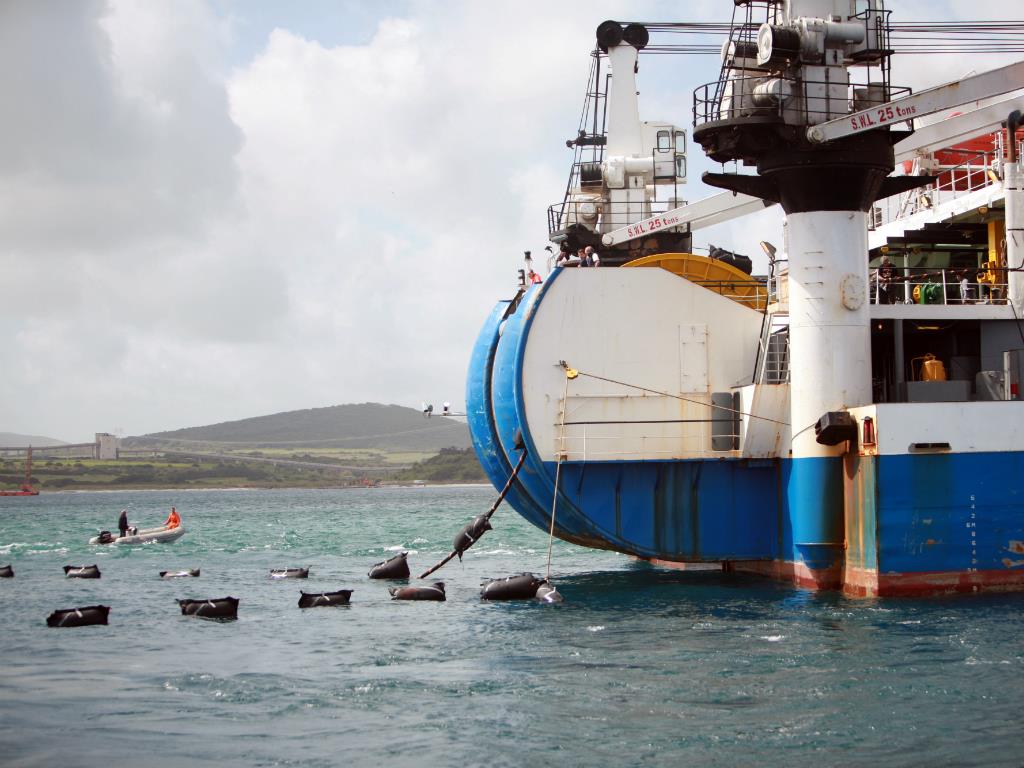This vibrant color photograph captures a distinctive ship, identified by its white hull adorned with blue stripes, anchored on a body of water, possibly a lake or the ocean. The vessel features a notable half-circle extension at its base, likely a piece of industrial machinery. Extending from this circular component into the water is a large rope. Outshining the ship's elaborate setup are two rows of plastic floats, aligned on the water to the ship's left, which give the appearance of marking a lane.

A vibrant scene unfolds as two individuals, dressed in orange and black, navigate a gray inflatable motorboat on the left side of the image. Both are likely part of a crew operating near the ship. Enhancing the detailed composition, rust marks on the ship hint at its sturdy, metallic construction, further characterized by various square shapes and substantial columns extending upwards. A white tower with cables and a series of levels and platforms populated by people are visible, adding to the complexity of the ship's industrial appearance.

In the backdrop, a hazy hill stretches across the horizon, dotted with patches of light green grass and clusters of dark trees. There's also a bridge subtly spanning part of the landscape. The sky overhead is predominantly cloudy, casting a diffuse light over the scene, creating a blend of industrial activity and serene natural elements.